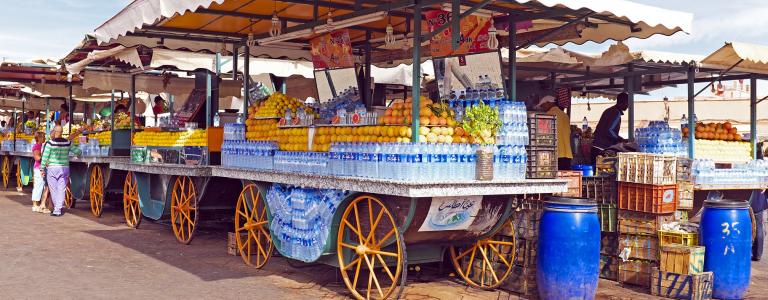The image, taken on a sunny, overcast day at what appears to be an outdoor marketplace, captures a horizontal line of nearly identical fruit carts stretching from the middle left to the upper right corners. The carts, each topped with small white awnings, feature large yellow wheels and are stocked with merchandise, including bottled water and various fruits—likely oranges, grapefruits, or lemons, due to their orangish-yellow hue. The central cart is viewed partially from the side and back, showcasing bottles and dark-colored crates. Blue barrels are positioned behind this cart and near more crates at the bottom right corner.

In the bustling scene, additional rows of carts fade into the distance on both the left and right sides of the image. Each cart is adorned with lights, calendars, and mirrors attached to their pillars. A person stands beneath the canopy of the central cart, and another nearby cart also has an individual inside. Two carts down, people walk along the street, seemingly tourists, engaging with vendors or perusing the displayed goods. The sky is visible in the corners, indicating the outdoor setting.